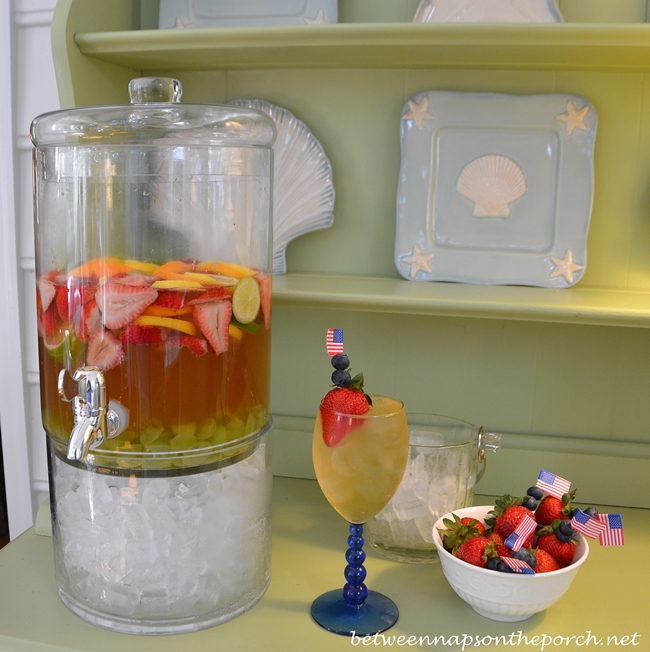This photograph, sourced from the website betweennapsontheporch.net as indicated by the watermark in the bottom right corner, showcases a meticulously styled scene centered around a faded olive green sideboard. The sideboard, which features shelves adorned with decorative baby blue plates showcasing shell motifs, presents a cohesive coastal theme. Prominently placed in the foreground is a large, clear drink dispenser containing an amber-colored beverage. The dispenser is layered with ice at the bottom, followed by sliced green grapes, and topped with floating slices of strawberries, lemons, oranges, and limes. To the right of the dispenser is a glass with a distinct blue stem, filled with the same amber liquid and ice, adorned with a floating strawberry, two blueberries, and a small American flag toothpick. Beside the glass sits a bowl filled with strawberries and blueberries, similarly decorated with miniature American flags. The attention to detail in the arrangement and the harmonious color palette contribute to a beautifully coordinated and inviting presentation.